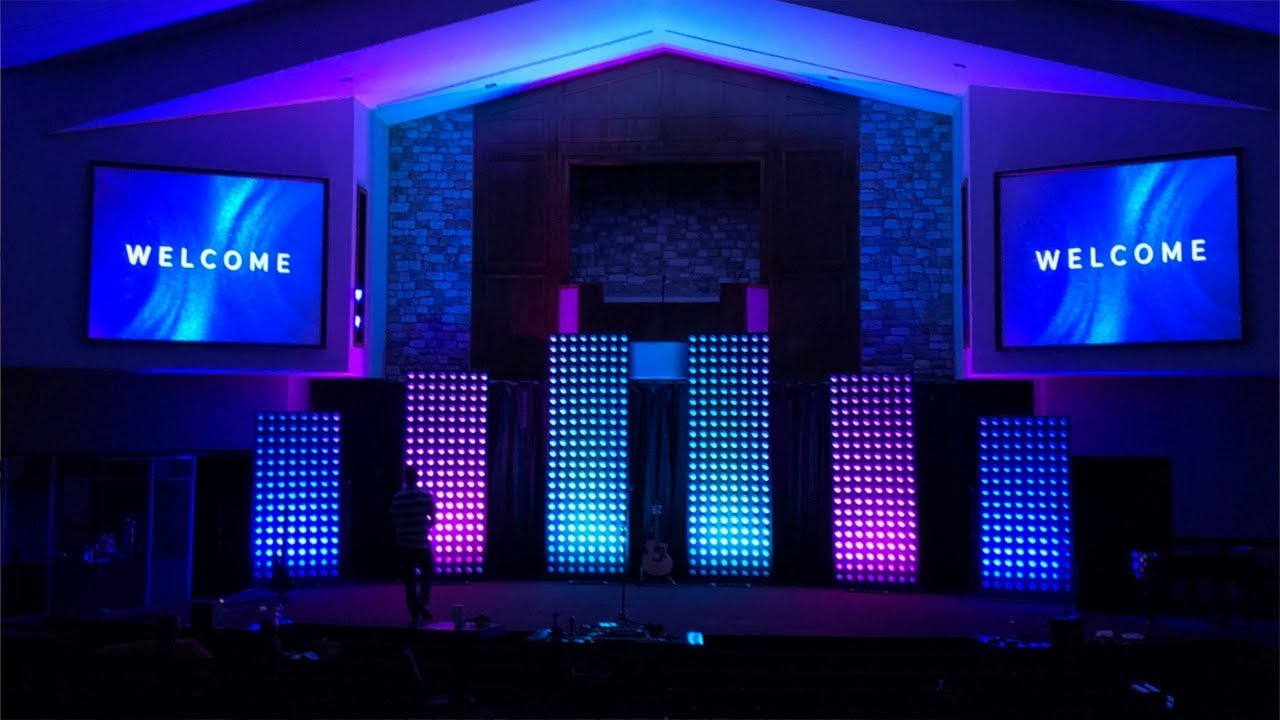The photograph captures an indoor auditorium bathed in an array of artificial lights, predominantly blue, red, green, and purple hues. The image, horizontally rectangular, shows a stage at the forefront adorned with six light stands, featuring an alternating pattern of colors: blue, red, and green. The ambiance is quite dim, with a significant portion of the lighting coming from these stands. 

At the upper center of the image is a distinctive archway with a white peak and brick sides, resembling a stylized home. This archway features various textures, including blue hues inside and brown wood framing the opening. Flanking this archway are two large display screens prominently displaying the word "WELCOME" in white capital letters against a blue background with white swirls.

The stage below is starkly lit, creating a contrast against the darkened auditorium. A person can be seen positioned on the left side of the stage, with faint outlines of an audience visible, indicating a likely performance setup. Additional elements such as a guitar and speakers enhance the stage’s setup, with some equipment possibly in preparation mode.

Overall, the venue exudes an atmosphere filled with vibrant colored lighting, inviting visuals, and architectural features that blend to form a compelling and visually intricate scene.